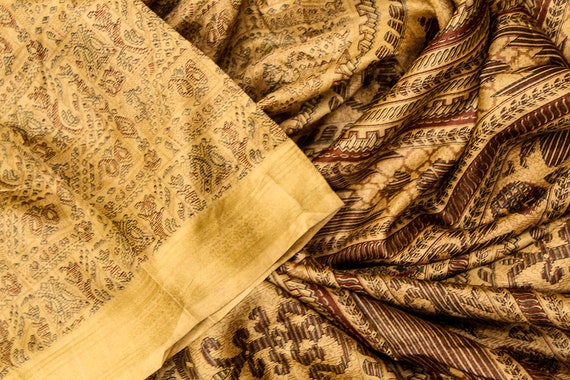This close-up image captures the intricate details of two overlapping, ornate pieces of fabric. The fabric on the left showcases a gold-on-yellow hem at the bottom, adorned with an extremely subtle pattern. Above this hem, the fabric features a delicate blend of light brown and red hues, forming an elaborate pattern of flowers, circles, crescents, dots, diamonds, and shapes resembling tree branches. The fabric on the right, in contrast, is richer and has a sheen to it, with a heavier texture. This fabric is marked with darker, deeper shades of rusty red and dark brown, presenting a more complex and bold pattern. The patterns on this fabric also feature a variety of shapes, including arrows, diagonal lines, frilly motifs, and floral designs. Overall, both fabrics exhibit a harmonious mix of intricate detailing and rich colors, with the left one emphasizing a more subtle elegance and the right one exuding a lavish and opulent appearance.